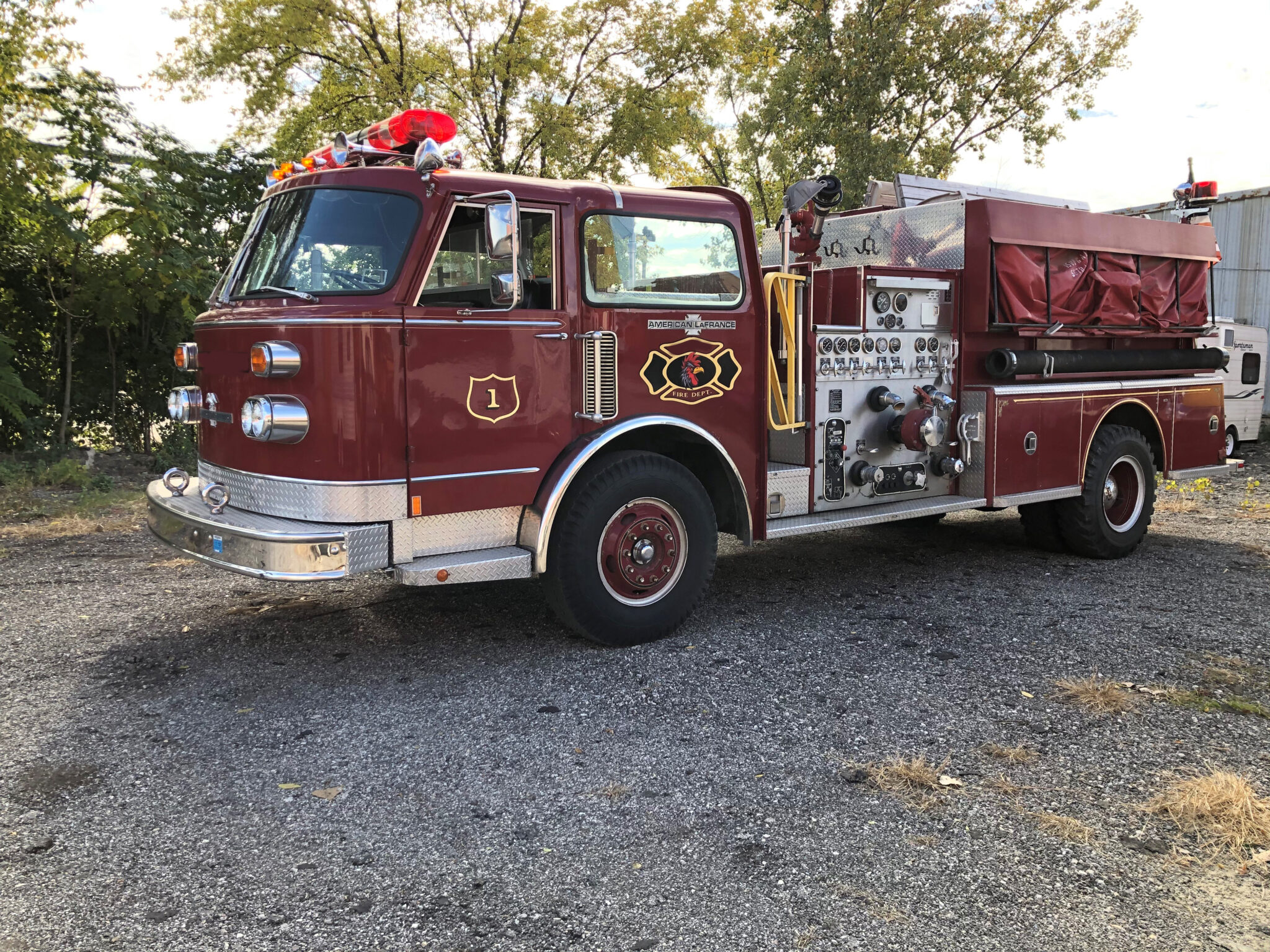This photograph captures a vintage fire engine, specifically fire engine number one, in a gravel parking lot that seems to be part of a small-town firehouse. The truck is a darker, muted red, almost maroon, rather than the typical bright red seen on modern fire engines. Likely built in the 1950s or 60s, this older model features a cab at the front with seating for the driver and an assistant, followed by additional seating capable of accommodating a crew of six to eight firefighters. Behind the cab, there is space for pumping equipment with various attachment points for hoses, and a storage box likely containing the hoses and other firefighting gear. The truck is adorned with a considerable amount of chrome and detailed gold accents, adding to its vintage charm. This functional yet classic firetruck, with all necessary gauges, lights, and sirens, seems well-equipped to handle firefighting tasks, potentially still in use by a rural fire station.